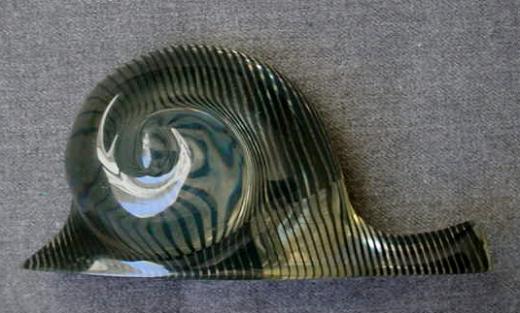This close-up photograph features a small, snail-shaped sculpture made from a material resembling either glass or hard plastic. The snail is predominantly black and gold, with intricate streaks of blue and white that spiral toward the center of its body, suggesting a sense of motion. The sculpture is highly reflective, with the thickest and most raised part of the design glinting under a light source. The flat base indicates it is designed to be displayed, likely on a shelf. The object is placed on a light gray fabric, possibly a tablecloth or couch cushion, which serves as the background. Additional hues, such as subtle blacks and grays, contribute to the overall aesthetic. The setting appears to be indoors.